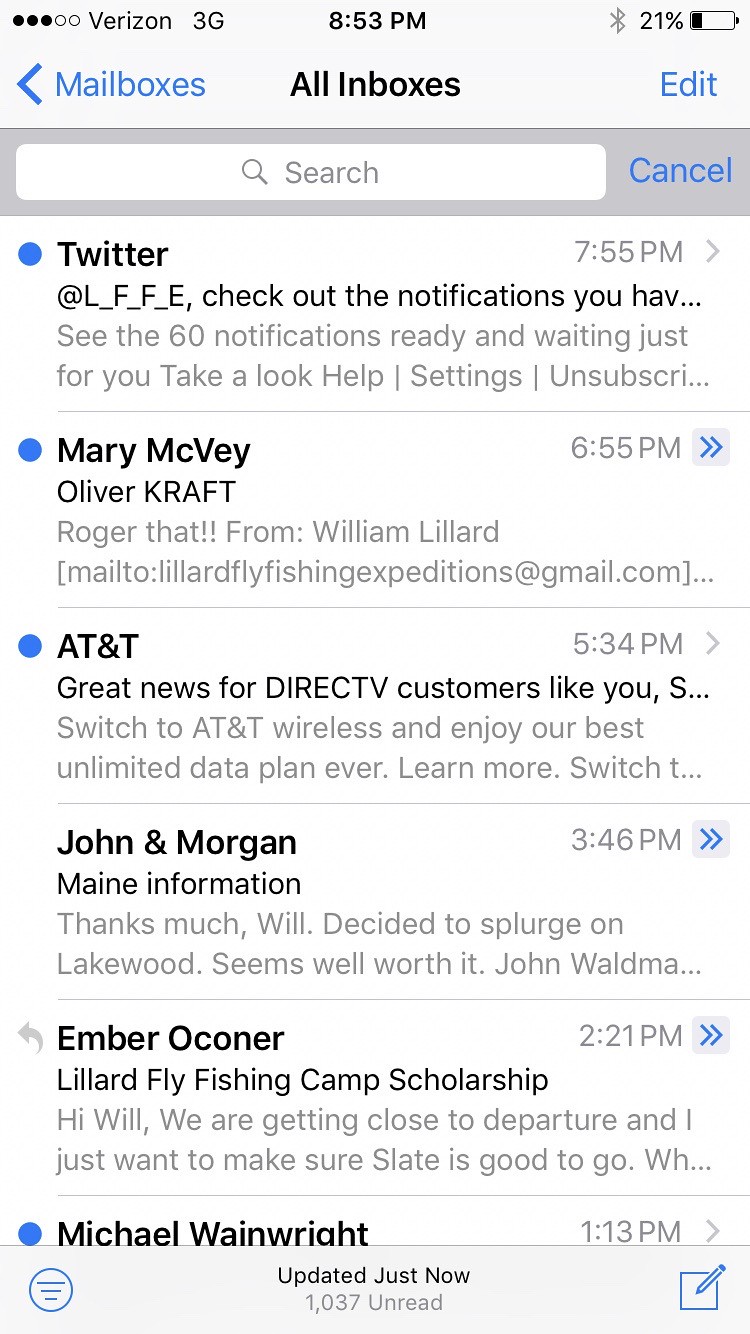The image captures a screenshot of an email app on an Apple device, displaying various levels of detail about the emails and the device's status. At the top, the status bar shows that the device is connected to Verizon 3G with three bars of signal strength, the time is 8:53 p.m., and the battery is at 21%. Below this, the header includes options for "Mailboxes," "All Inboxes," and "Edit." 

Next, there's a search bar with a magnifying glass icon on the left and a "Cancel" button on the right. Following that, the screen displays a series of email headers. The first email is from Twitter, sent at 7:55, with a blue bullet point indicating it is unread, inviting the user to check out 60 notifications. The second email is from Mary McVeigh, received at 6:55, stating "Roger that," also marked with a blue bullet. The third email, from AT&T, arrived at 5:34. The fourth email is from John and Morgan, received at 3:46, mentioning they decided to splurge on Lakewood. Next is an email from Ember O'Connor about a fly-fishing camp scholarship, sent at 2:21. The final listed email is from Michael Wainwright. 

At the bottom of the screen, it notes that the email list was "updated just now" with 1037 unread emails. Each email header includes subtext previewing the content and corresponding timestamps. Blue arrows in a silver box are visible next to some emails, indicating additional options or actions.